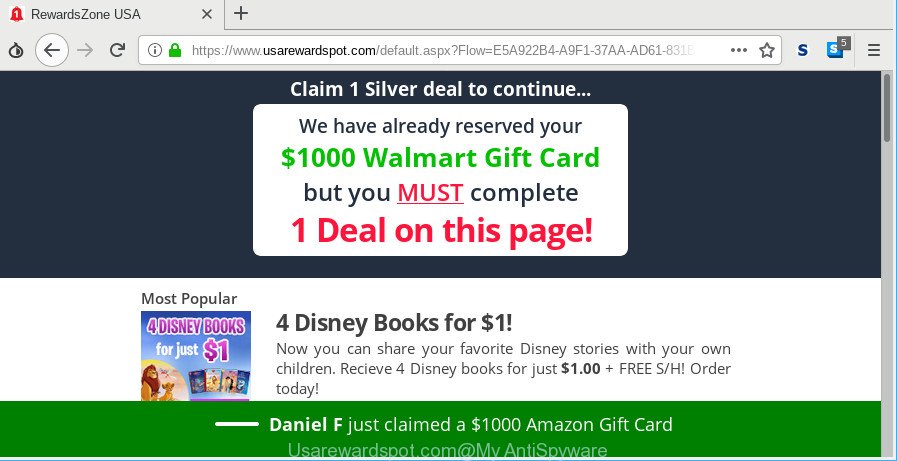In the image, we see a screenshot from the website "USA Reward Spots" (https://www.usarewardspots.com/). The top-left corner features tabs such as "Reward Zone USA" with an "X" to close and a plus sign adjacent to it. Below these, there's a circle icon with a left arrow for navigation, a reload icon, and a search bar starting with an "I" enclosed in a circle. A secured connection is indicated by a green closed lock icon next to the website URL, which reads "https://www.usarewardspots.com/default...". 

At the end of the address bar, there is a bookmark star icon. Below this, a prominent black rectangular box displays the message "Claim one silver deal to continue." Within a highlighted white box, the text "We have already reserved your $1,000 Walmart gift card, but you must complete one deal on this page." stands out, with "one deal on this page" in red and an exclamation mark, and "must" underlined and in capital letters for emphasis.

Towards the lower portion, under the heading "Most Popular," there's an offer featuring "Four Disney books for $1." Users are prompted to claim this deal by pressing the green button provided.